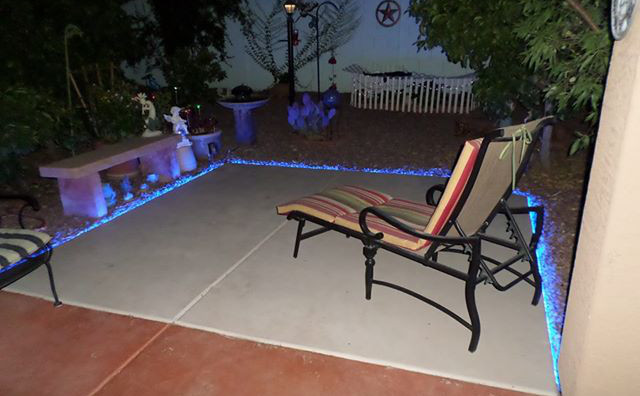The photograph depicts an outdoor patio area, possibly a porch or backyard, taken either in the evening or nighttime. The rectangular image, about four to five inches wide and three inches high, showcases a space with distinct flooring sections. The lower left portion features light orange, reddish cement tiles, while the central and right parts are covered in gray poured concrete blocks. Surrounding the concrete area, blue LED lights with purple tips add a touch of color.

On the right side of the patio, there's a black-framed lounge chair with a striped cushion in shades of yellow, red, green, and beige. In front, the patio is bordered by light-colored gravel and mulch, adding texture to the scene.

In the background, a white wooden fence stretches across, adorned with a red star inside a circle. To the left and right of the patio area, trees and plants add greenery, and a concrete stone bench sits on the left side. Additionally, there appears to be a white wall on the right side of the image, framing the patio area. A round fountain or birdbath adds a final touch to the picturesque outdoor space.